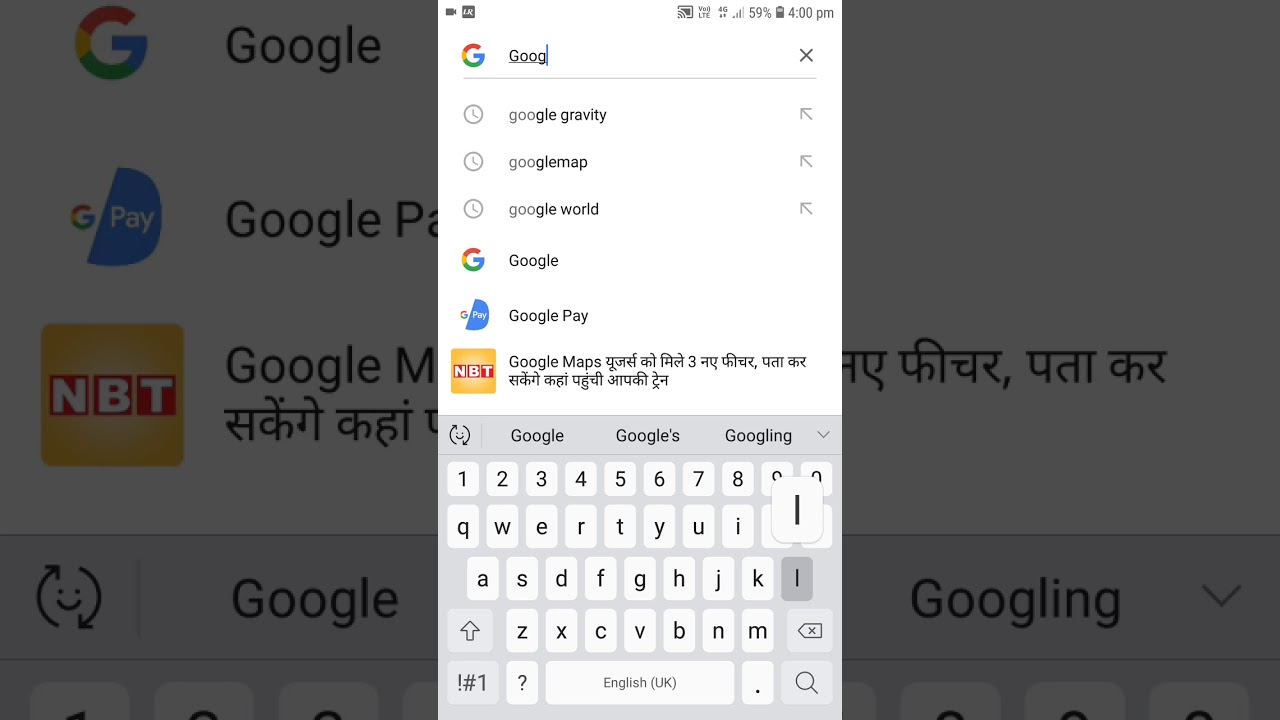This composite image features two distinct sections. The bottom section is lightly obscured by a gray overlay, making the text somewhat difficult to decipher. In the top left corner of this bottom section, the image includes a small 'G' logo followed by the word "Google." Directly beneath this, there is the Google Pay logo, next to which one can make out the words "Google P," though the rest of the text is blocked by an overlay.

Below the fragmented "Google P" text, there is a yellow square containing the letters "NBT," accompanied by the word "Google" and the letter "M," with the rest of the text cut off. Below this, there seems to be text in a foreign language, followed by a smiley face encircled by two arrows.

The overlay on the bottom section is, in fact, another image resembling a cell phone screen with a white background. At the top of this screen, we see the Google logo with the text "G-O-O-G" and a cursor positioned after the last 'G'. Beneath this are three entries, each preceded by a clock icon. The first entry reads "Google Gravity," the second "Google Map" (written as one word), and the third "Google World." 

At the bottom of the phone screen image is a virtual keyboard displaying a standard QWERTY layout. The top row includes numbers 1 through 0, and the space bar at the bottom is labeled "English UK."